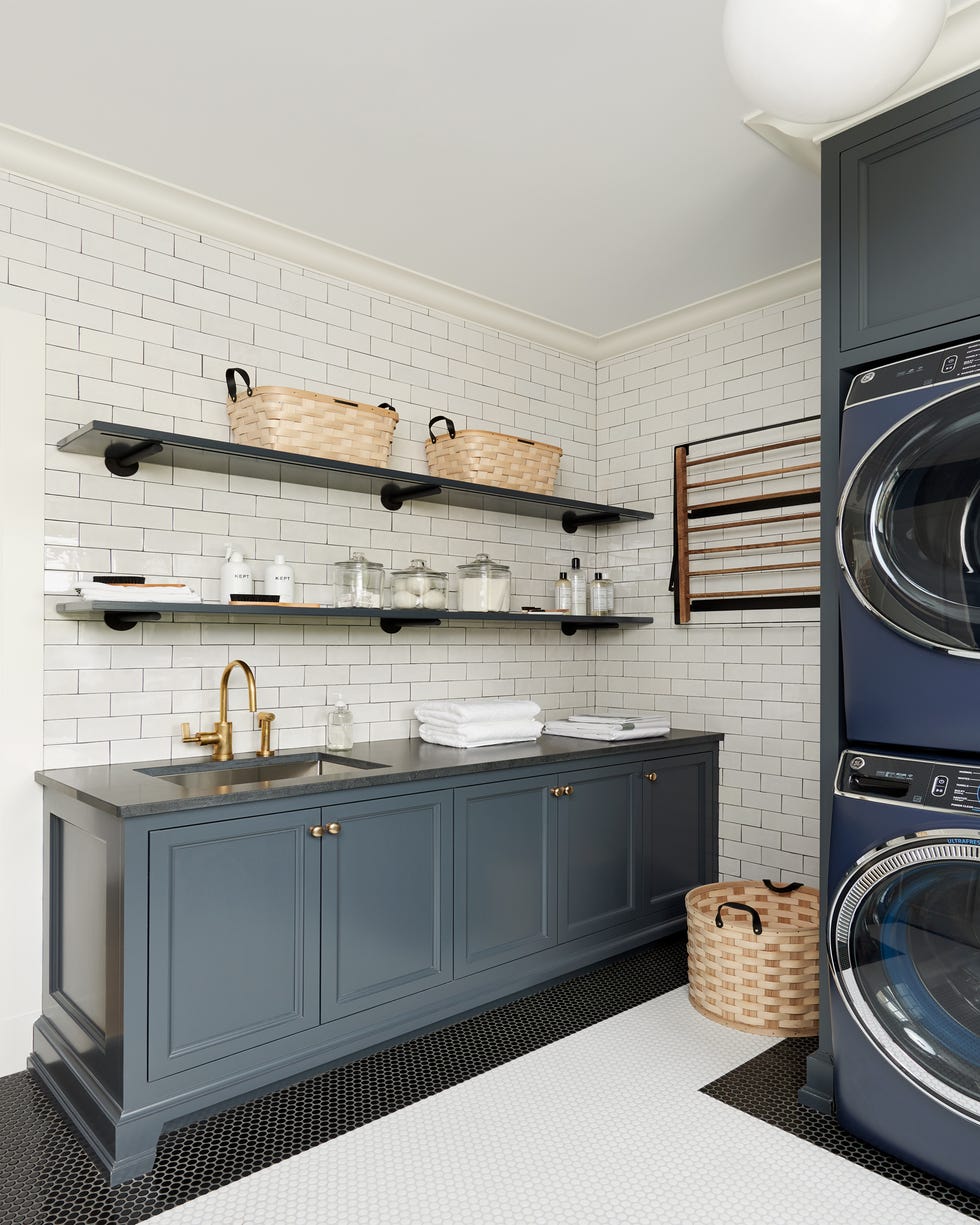The image depicts a modern, well-appointed laundry room featuring white rectangular tiled walls and small hexagonal white and black floor tiles. To the right side of the photo, there is a navy blue washer and dryer set stacked vertically, seamlessly integrated into matching cabinetry. Centrally, a countertop with a gold-handled sink is flanked by dark blue, almost gray, cabinets. Above the sink area, two shelves are positioned: the top shelf holding two light wooden baskets, and the lower shelf lined with an assortment of glass jars and bottles. The countertop itself hosts a couple of neatly placed towels, and to the left of the washer and dryer, a sizable woven basket rests on the floor. The room's layout and design elements, such as the cohesive cabinetry and well-organized storage, contribute to its functional yet stylish ambiance.